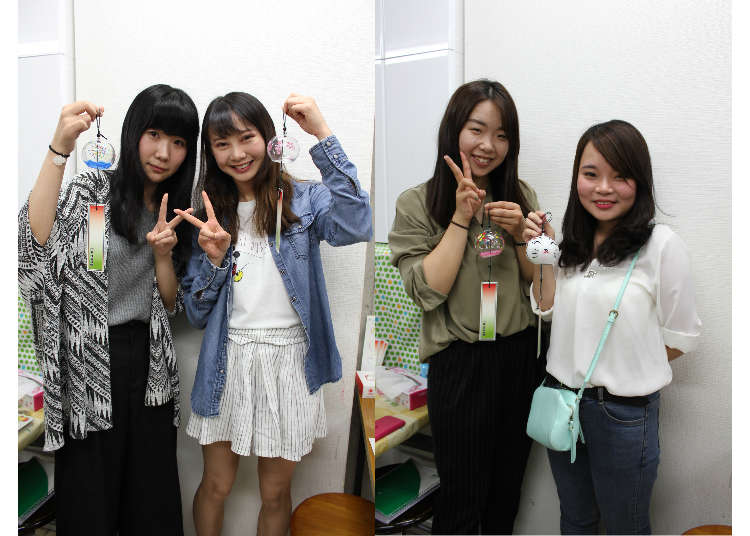This detailed color photo features two groups of young Asian girls in their early teens, captured in adjacent images. Each photo showcases two girls, together making a total of four. All four girls have dark hair—two with black and two with brown. In both photos, the girls are flashing peace signs and holding small, transparent, spherical charms. The backgrounds feature green and orange dotted patterns on paper.

In the left image, the first girl on the far left is dressed in a black dress and a gray and white shawl, while the second girl wears a white striped short dress paired with an unbuttoned denim jacket. Both girls are holding small, transparent, pumpkin-shaped charms.

In the right image, the third girl is clad in an olive green shirt and black pants, with an accessory on her right wrist, while the fourth girl sports a white blouse and medium blue jeans. One of the charms in this image is described as having a face resembling a white cat. The walls behind them are predominantly white with black at the bottom, and the scene displays an array of colors including blue, white, green, orange, yellow, and red.